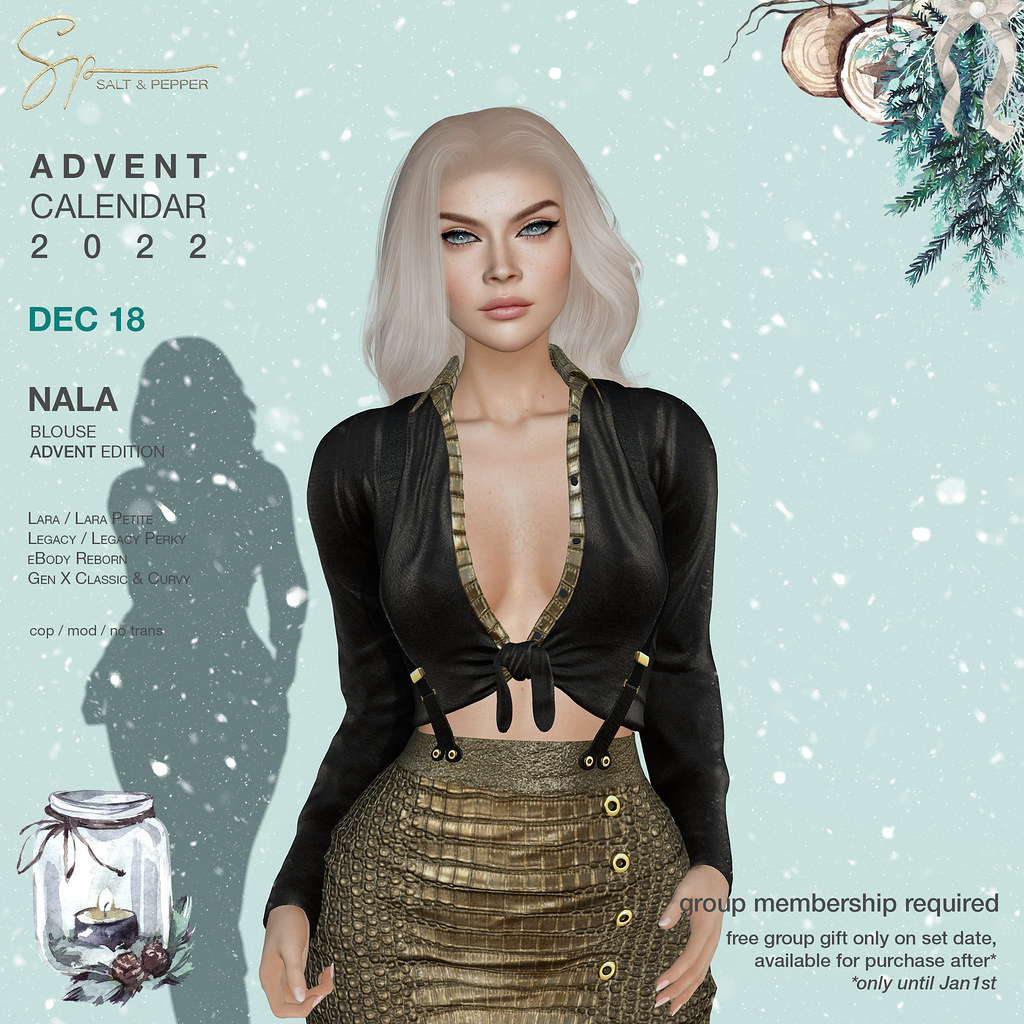The image is a detailed digital rendering of a fair-skinned woman with shoulder-length, wavy white hair and very light gray-blue eyes, wearing makeup. She is dressed in a black leather-looking top with a plunging neckline that reveals some cleavage, and a tight-fitting golden bronze snakeskin skirt. The background is light teal with white snowflakes scattered throughout, enhancing the festive theme. At the top, Christmas ornaments and evergreen branches with pine needles and a bow are displayed, adding to the holiday spirit. The top left corner features a gold metallic logo that reads "Salt and Pepper," along with the text "Advent Calendar 2022 December 18 Nala Blouse Advent Edition." Additional text to the left includes: "Lara/Lara Petite, Legacy/Legacy Perky, eBody Reborn, Gen X Classic and Curvy, Cop/Mod as Copy/Modify/No Transfer." Below the main image, there's a glass jar with a candle graphic, and in the bottom right, text indicates "Group membership required, free group gift only on set date, available for purchase until January 1st."